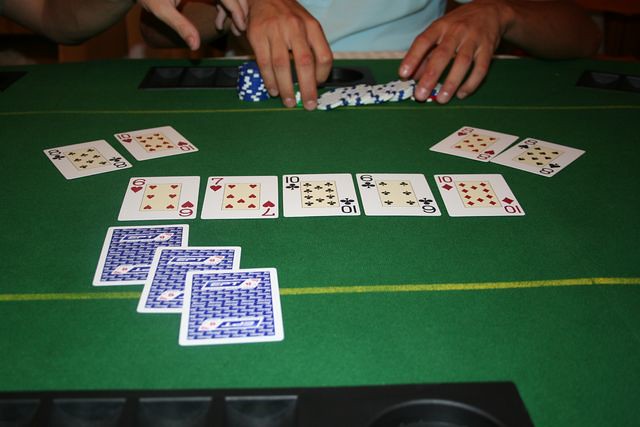In this close-up image of a high-stakes poker game, the vibrant green felt table sets the stage for an intense match. At the center of the frame, a row of community cards reveals a dramatic spread: 6 of hearts, 7 of hearts, 10 of clubs, 6 of clubs, and 10 of diamonds. On either side of these cards, pairs of upturned cards create additional intrigue; the left side showcases the 8 of clubs and 10 of hearts, while the right side displays the 8 of hearts and 8 of spades.

In the foreground, three blue and white face-down cards maintain a sense of mystery, concealing their values. Accompanying these cards is a sleek black tray designed to hold poker chips. Further into the background, the hands of a Caucasian man are diligently stacking white and blue chips, indicating a likely winning hand or a strategic bluff. Nearby, an enticing stack of bright blue chips with white accents draws the eye. Adjacent to his hand sits another black chip tray, adding to the organizational setup of the table.

In the upper left corner of the image, another Caucasian hand reaches down toward the stack of dark blue chips, suggesting an imminent move. The composition of elements in this photo paints a vivid picture of the high-energy, calculated world of poker.